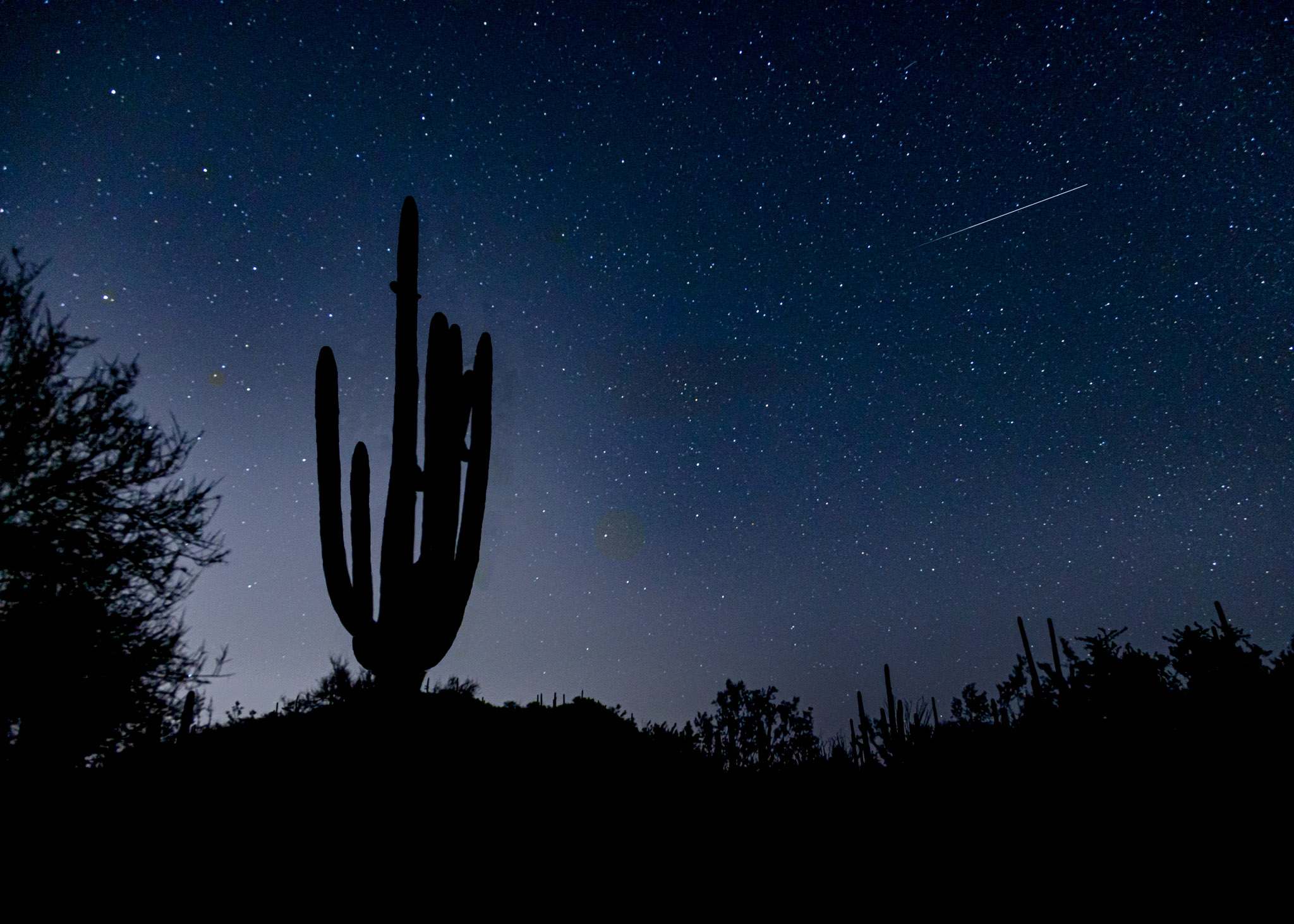This image captures a serene outdoor landscape at night. The bottom portion of the photograph reveals a dim, uneven ground dotted with various plants, all appearing as black silhouettes. Among these, a prominent cactus with six distinct stems is clearly visible on the left side, accompanied by the delicate, thin leaves of a tree. The night sky above is a deep, dark blue, slightly brightened at the bottom left corner, and studded with numerous dot-shaped, white stars. A striking feature of the sky is a shooting star, seen as a white line streaking upwards towards the right corner. The overall scene is one of stark contrasts, with the inky black shapes of the plants against the tranquil, starlit sky.